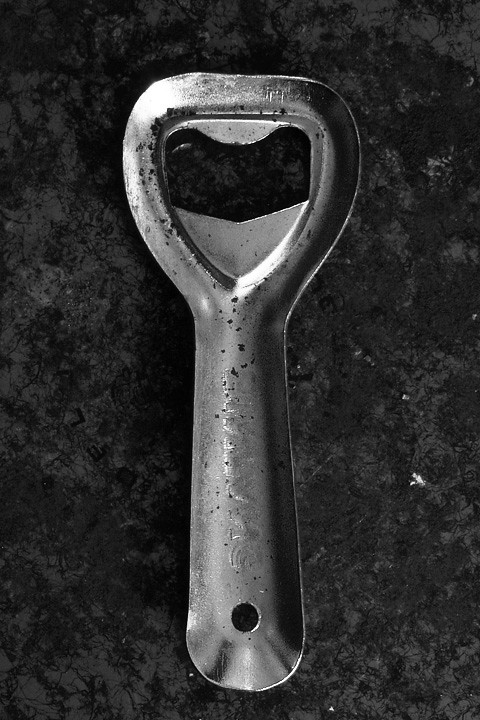The image depicts a small, aged metal bottle opener with a heart-shaped top. The opener, primarily silver in color but tarnished with numerous black dots and scratches, appears well-used. Positioned on a black, granite-like surface sprinkled with white speckles, the tool features a rounded end with a circular hole, likely for hanging. The handle, which looks thin and not particularly ergonomic, shows remnants of old, unreadable writing. The bottle-opening mechanism includes a rounded part for gripping the bottle cap and a thin metal piece beneath with a slight V shape for prying off caps. Despite its rustic appearance and visible wear, the opener remains functional and is prominently centered in the image.